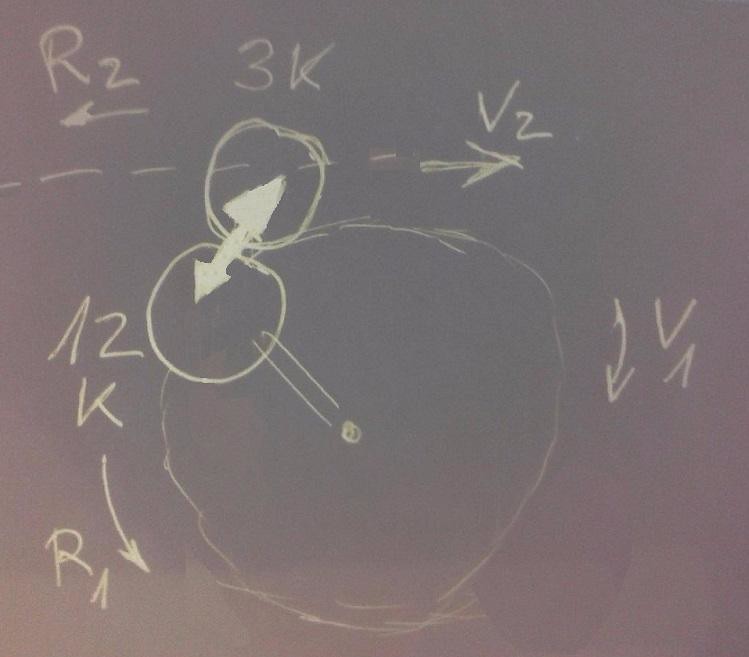The photograph captures a grainy, analog-style image of a chalkboard filled with a complex series of diagrams and annotations. The composition appears to illustrate either a scientific formula or a set of instructional steps. 

In the upper left corner, there is a capital "R" followed by a subscript "2" (R₂) with an arrow pointing left, beneath which another arrow is located. To the right, the notation "3K" is placed. Below these elements, a dashed arrow extends horizontally to the right, terminating at the label "V₂." 

Central to the diagram is a circular structure that seems to represent a cyclical process, segmented by a Venn diagram suggesting diverging paths. Various other labels such as "A₂," "K," "R^" (capital R with a caret), and "V^" (capital V with a caret) are scattered throughout, accompanied by random chalk arrows, adding to the intricate and somewhat chaotic layout of the chalkboard.

The grainy texture and old-school feel of the image, likely due to the use of an analog camera or an intentional flash effect, lend the photo an extra layer of vintage authenticity, capturing the essence of a bygone academic era.